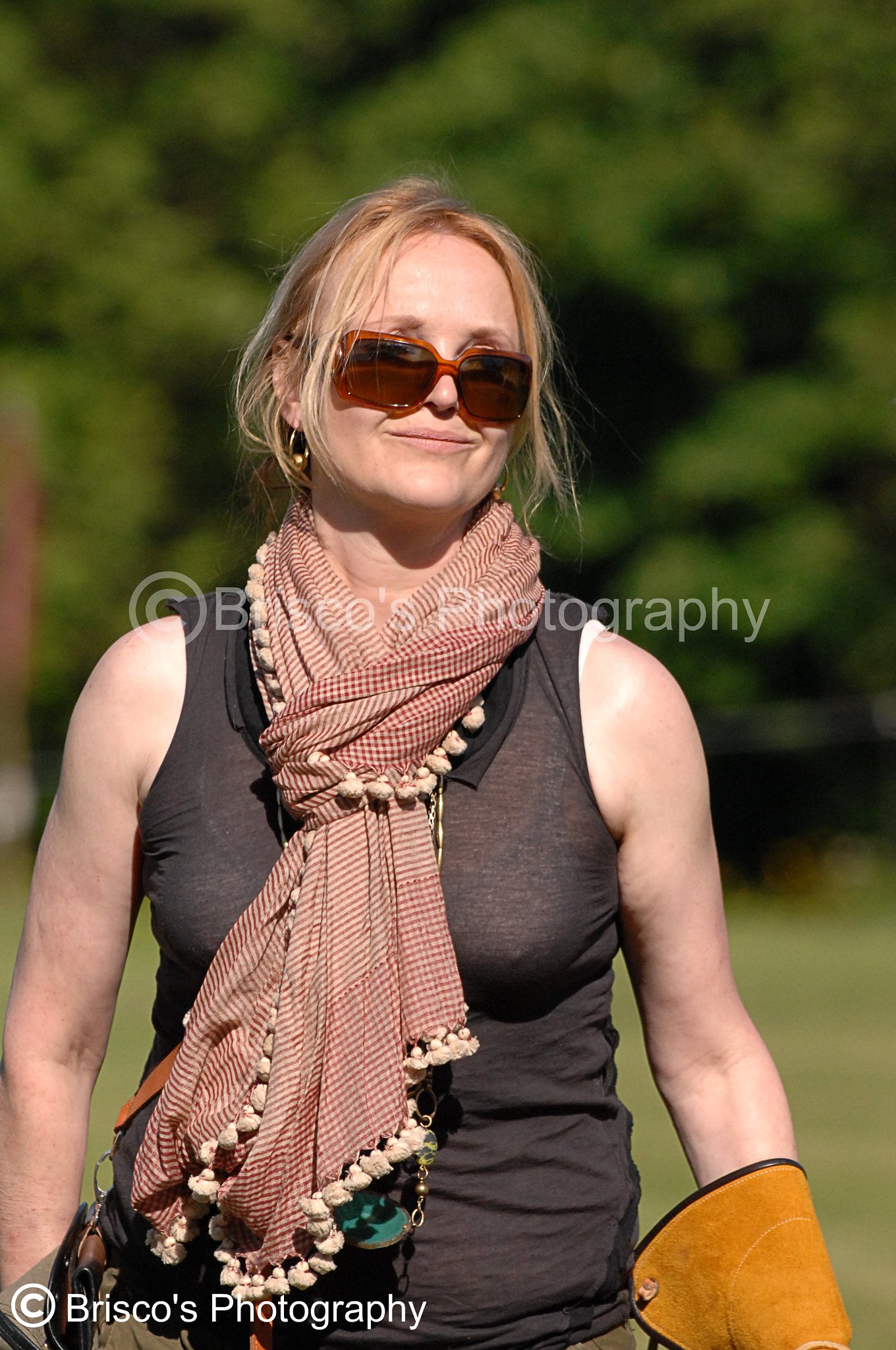This is a detailed color photograph of a woman in her 30s, taken by Briscoe's Photography, with watermarks superimposed in the center and at the bottom left of the image. The background features blurred green trees and grass, emphasizing the woman as the main subject. She has light brown hair pulled back and wears gold dangly earrings. Her eyes are partially covered by red octagonal sunglasses perched low on her nose. She is smiling subtly, not showing teeth.

She is dressed in a black or gray, very thin, almost see-through tank top, with her arms exposed. Around her neck, she sports a red checkered scarf with white fringe. On one arm, she wears a distinctive tan leather glove that extends to her elbow, while the other arm appears to be partially cropped out of the image. The overall scene suggests a sunny day, adding a bright and cheerful atmosphere to the photograph.